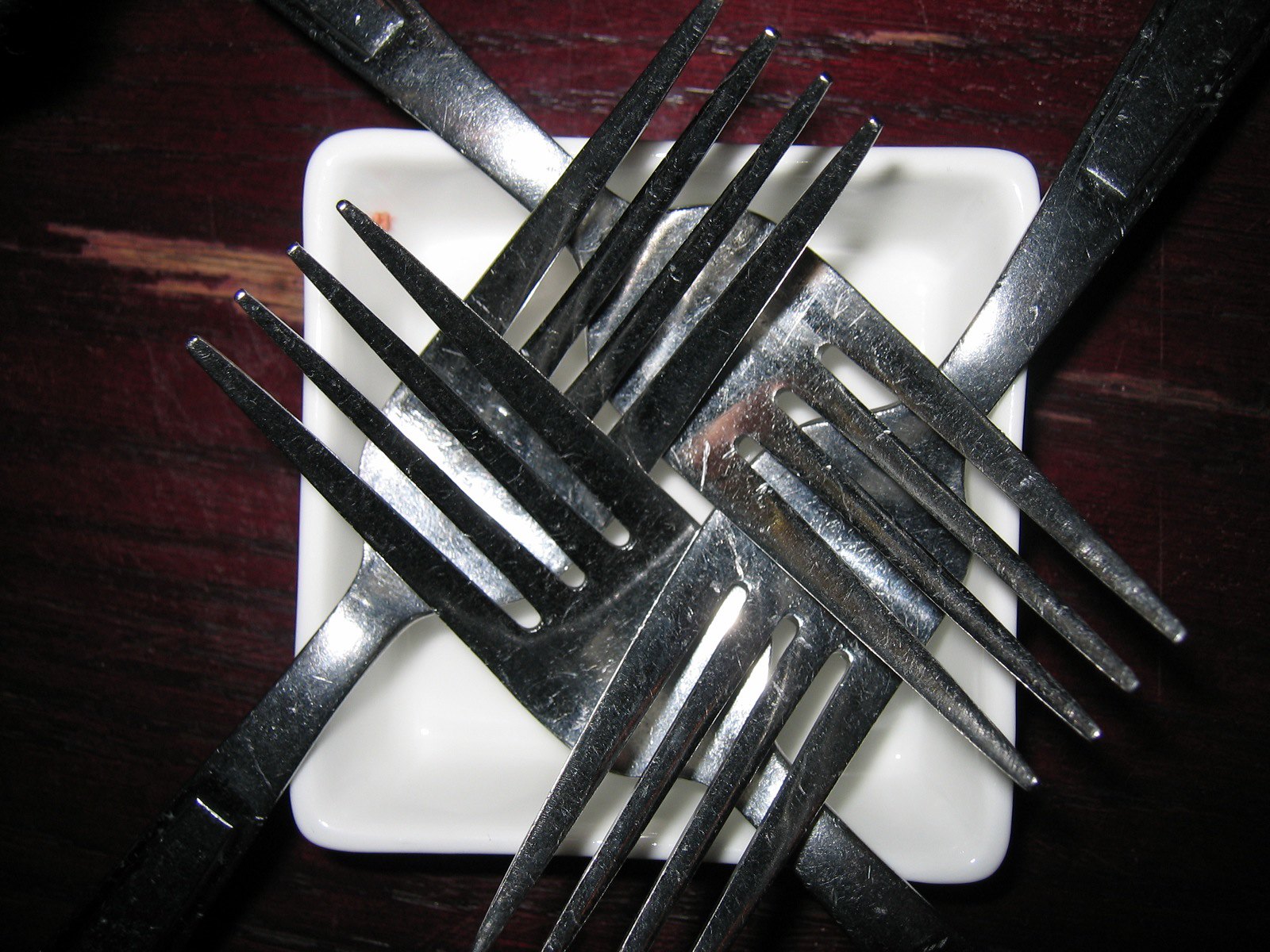This top-down photograph captures a close-up view of four well-used silver forks arranged in a swastika-like pattern, with their tines touching to form a square in the center. The forks are placed on a small, reflective white square plate, possibly made of plastic or porcelain. The image is taken against a deep red, distressed wooden surface, likely mahogany. The zoomed-in perspective focuses on the forks' tines and partially shows their handles, which are marred with various nicks and scratches, indicating frequent use. The symmetrical, crisscrossed positioning of the forks creates an intricate, visually striking composition.